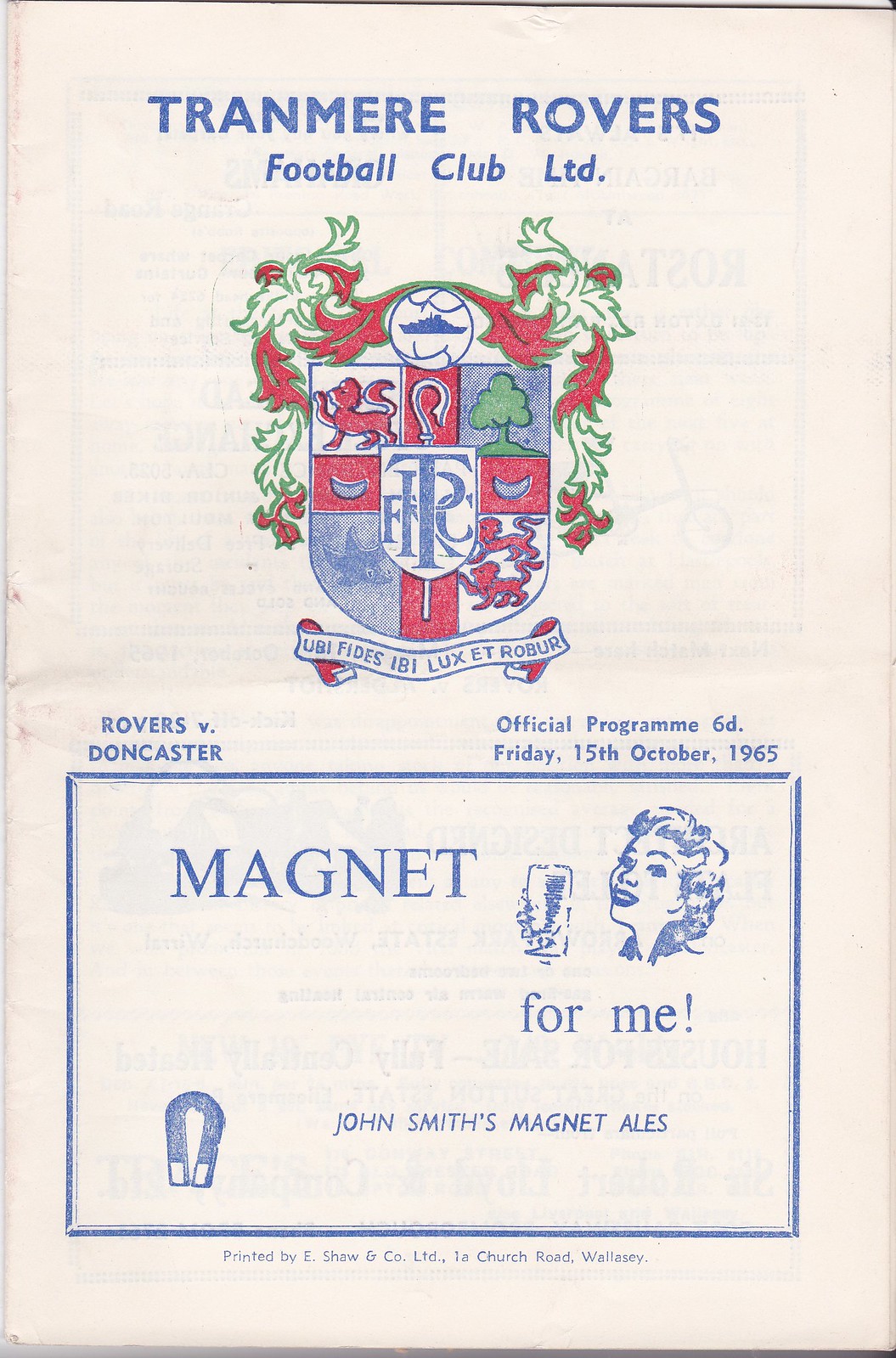The cover of this official program for a soccer game between Tranmere Rovers and Doncaster, held on Friday, October 15th, 1965, is straightforward and richly detailed. Set against an aged white background, the top of the cover features the text "TRANMERE ROVERS" in bold blue capital letters, followed by "Football Club Limited" in italicized blue text. Beneath this title, a large, detailed crest is prominently displayed. The crest, shaped like a shield, includes intricate elements such as a lion, trees, a bow within a soccer ball at the top, and the intertwined letters "TRFC" in the center. Below the crest, the text "Rovers v Doncaster" appears on the left side, while "Official Program 6D, Friday 15th, October 1965" is placed on the right. The lower portion of the cover features an advertisement within a blue-outlined rectangle. Inside, in blue text, the word "MAGNET" is positioned on the left, accompanied by a cartoon-style image of a woman lifting a pint glass on the right, with the slogan "for me!" Following this, at the bottom of the rectangle, the text reads "John Smith's Magnet Ales," flanked by a horseshoe-shaped magnet illustration, maintaining the vintage, minimalist aesthetic of the cover.